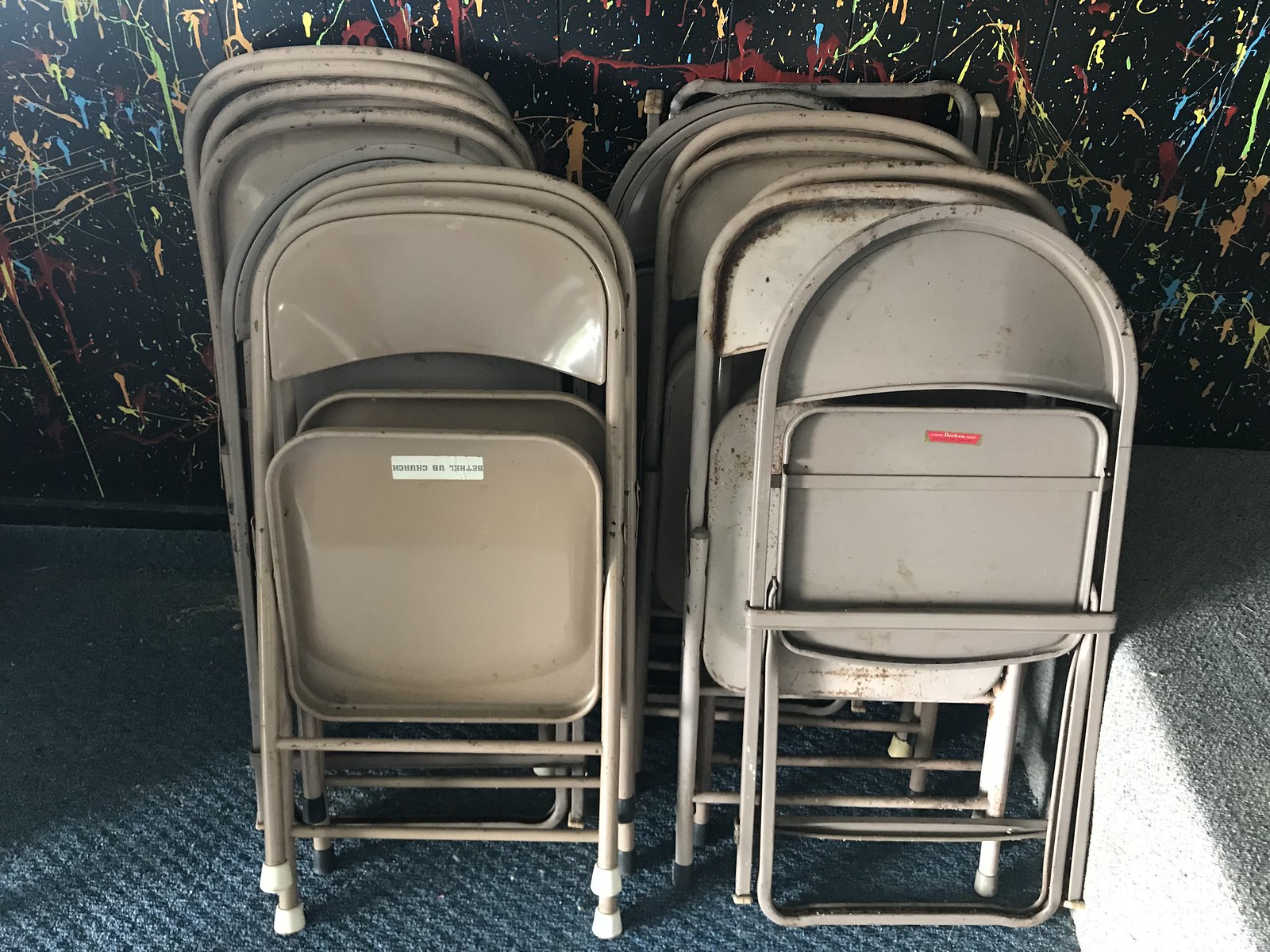The image portrays a stark, abstract scene dominated by a sprawling black wall that's whimsically splattered with paint in a myriad of colors, including blue, yellow, green, red, pink, lime green, and gold. The paint appears to be haphazardly thrown and allowed to drip and dry, creating a chaotic yet striking backdrop. In front of this colorful wall, there are about a dozen metal folding chairs, some leaning and some stacked in two uneven rows. The chairs vary in condition and appearance; some are newer with white caps on their legs and undamaged metal, while others are older and rusted, bearing signs of extensive use. The chairs also differ slightly in design, with some having rounded tops and others more squared. On the floor, a blue carpet complements the industrial feel of the setting, accompanied by a concrete step situated to the right. The overall scene suggests a past event or gathering, now left in a state of artistic disarray.